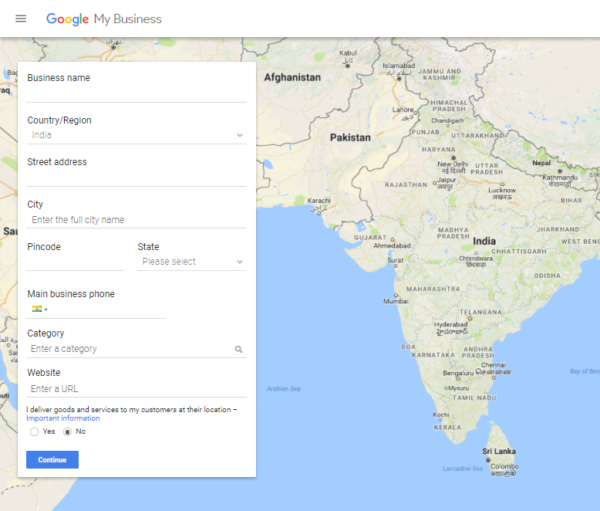This is a detailed screenshot of a Google My Business page displayed on a webpage. Positioned at the top left corner are three vertical lines, the Google logo in its recognizable colors, followed by "My Business." The background showcases a detailed map encompassing regions of India, Pakistan, and Afghanistan, bordered by the Arabian Sea on one side and a bay on the other. Sri Lanka is also visible, adding to the geographic context. The map features a palette of green, blue, orange, yellow, and light tan, with all text rendered in black, varying in boldness for emphasis.

A prominent white box on the left-hand side appears to be a form interface. The top field is labeled "Business name," inviting users to input relevant details. The following fields include "Country/Region" pre-filled with "India," "Street address," "City," "PIN code," and "State," which has a drop-down menu for selection. Additional fields request the "Main business phone" accompanied by a yellow and green icon, "Category," and "Website." Below these, a checkbox option indicates whether the business delivers goods and services to customers at their location, marked by "Important information" with a yes or no choice. At the end of the form, a "Continue" button is available for proceeding with the entry.